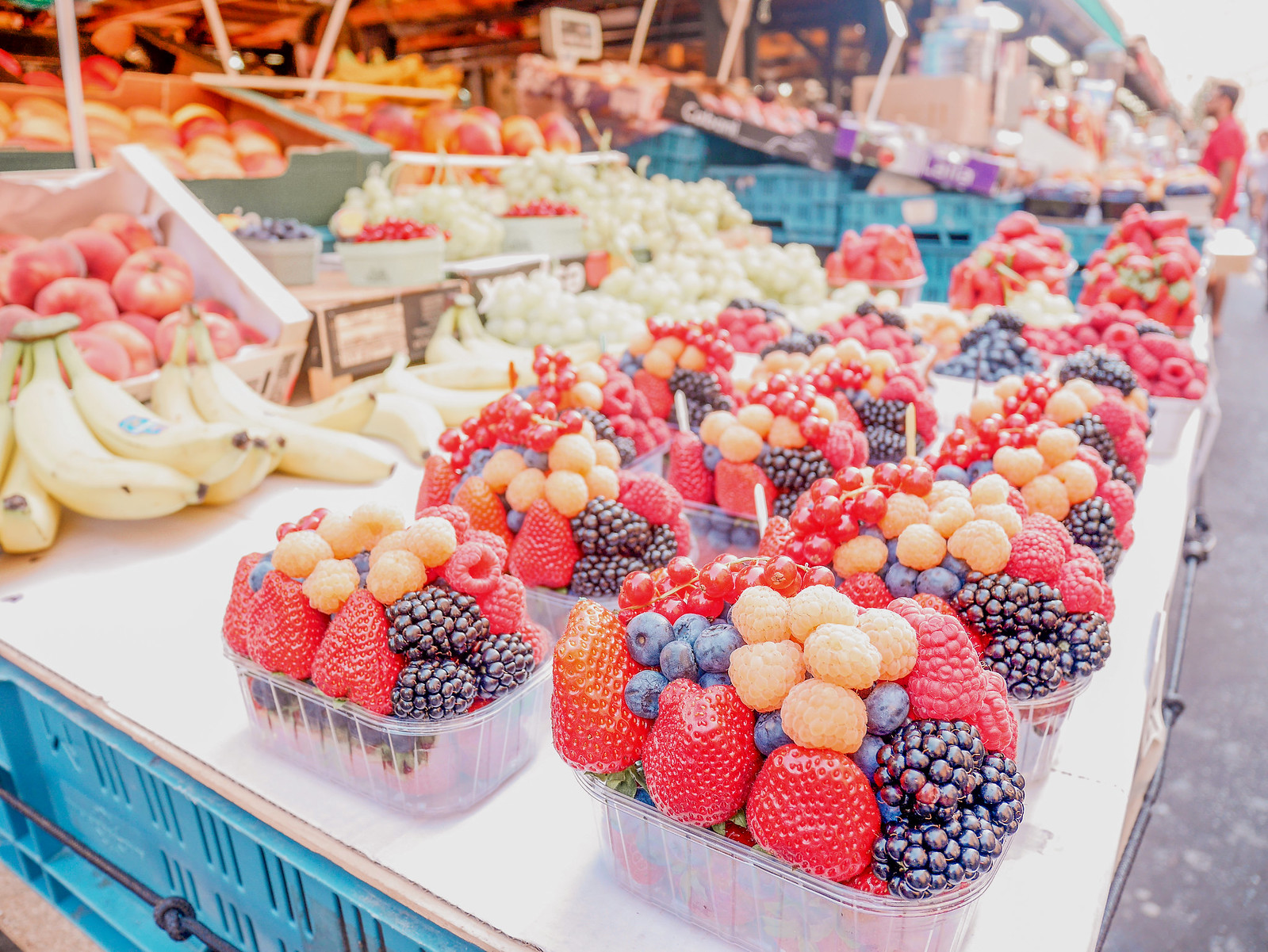The vibrant outdoor scene captures a dynamic angle of a bustling farmer's market. The perspective offered starts from the lower left-hand corner and follows a table laden with produce, stretching diagonally towards the upper right-hand corner, parallel to a street or roadside setting. The table is brimming with an array of clear plastic containers, overflowing with an assortment of fresh fruits. 

These containers are so abundant with produce that the fruits, which include strawberries, blueberries, blackberries, black raspberries, and some intriguing orange-colored berries similar in size and abundance to raspberries, seem precariously piled higher than the containers themselves. Behind these fruit-laden baskets, bananas and tomatoes are also visible, contributing to the tablescape that extends into the background, densely packed with produce.

The overall picture is extremely colorful and vibrant, hinting at the meticulous effort that went into arranging the baskets. The scene encapsulates the energy and variety typical of a farmer's market, showcasing a rich display of fresh, colorful fruits and vegetables in a lively outdoor setting.